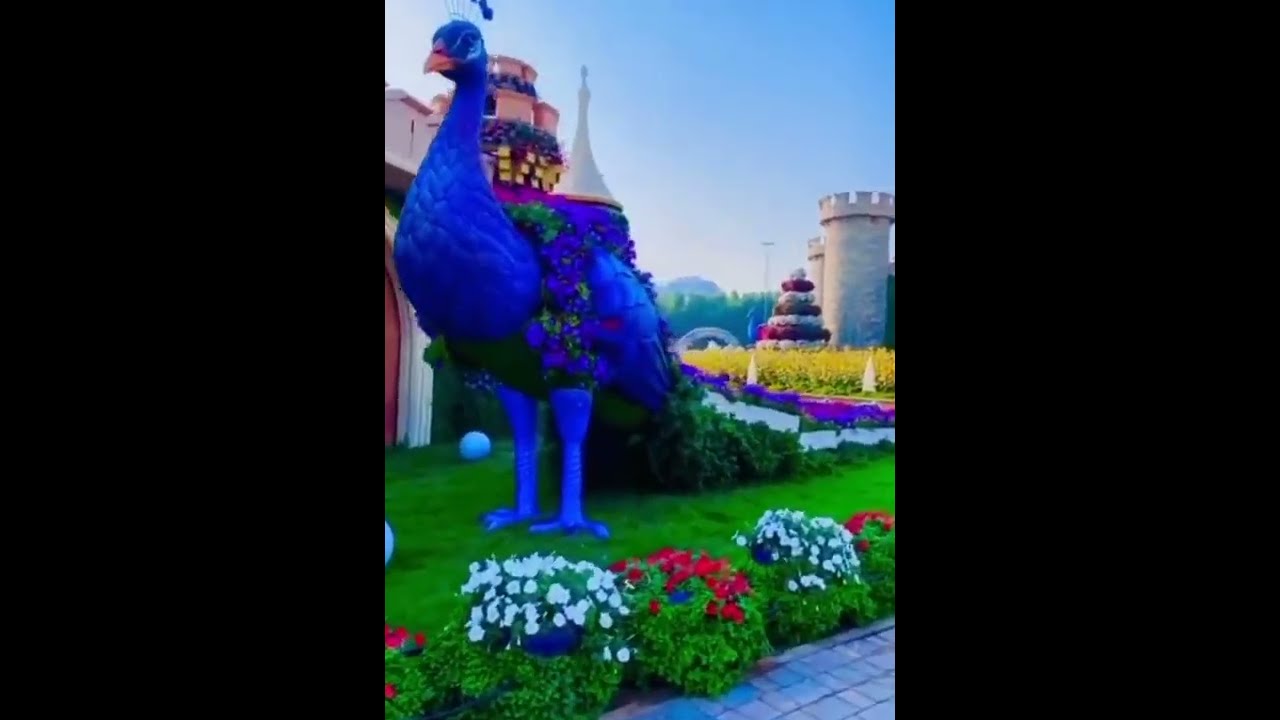The image depicts a vibrant, fantasy-themed scene, reminiscent of a theme park, possibly akin to Disney or Universal Studios. Central to the composition is a ginormous peacock statue adorned in striking blue with an elaborate tail made from red, white, and yellow flowers. This towering ornament is set amidst a lush green lawn, sprinkled with vivid floral arrangements in shades of red, white, purple, and yellow. The peacock is flanked by a stone path lined with meticulously maintained bushes of red and white flowers. In the backdrop, there are visually enchanting castle towers, one pink with accents of yellow and purple, and another white with tiered lavender elements, emphasizing the fairytale atmosphere. The sky is a flawless blue, perfectly clear of clouds, adding to the surreal, almost animated feel of the scene. The overall impression is that of a meticulously designed amusement park or elaborate mini-golf course, bursting with bright colors and whimsical decorations.